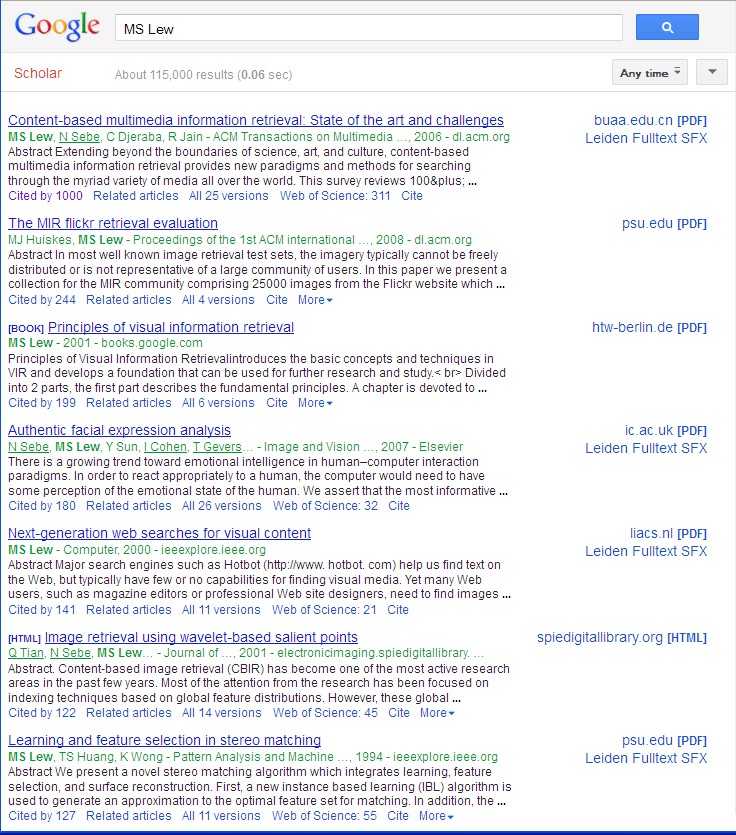The image depicts a Google Scholar search results page. In the top left corner, the Google logo is visible. Adjacent to it is a long rectangular search bar containing the text "MS LEW." To the right of the search bar is a blue square with a magnifying glass icon inside it. Below the search bar, "Scholar" is written in red text. The search results indicate about 115,000 results found in 0.06 seconds.

The results are categorized and underlined in blue, making them clickable links. The categories include:

1. **Content-Based Multimedia Information Retrieval: State of the Art and Challenges**
2. **The MIR Flickr Renewal Evaluation**
3. **Principles of Visual Information Retrieval (Book)**
4. **Authentic Facial Expression Analysis**
5. **Next Generation Web Searches for Visual Content**
6. **Image Retrieval Using Wavelet-Based Salient Points**
7. **Learning and Feature Selection in Stereo Matching**

Additionally, below these categories, there is information in green text displaying the authorship: "MS Law, T.S. Hong, K. Wong," followed by the publication source and year, "Pattern Analysis and Machine, 1994, IES Explore."